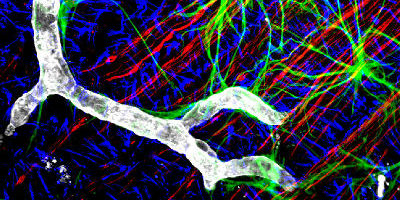The image is an intricate and abstract piece set against a black background, showcasing a vibrant array of colors and shapes that evoke both artistic and scientific themes. Dominating the composition are bold, bright lines in red, blue, and green, arranged in chaotic yet structured patterns. In the upper section, green lightning bolt-like lines radiate from a central point, creating an explosive visual effect. Red lines streak diagonally from the upper right to the middle and lower parts of the image, intersecting with the ever-swirling and zigzagging blue lines.

A white, branch-like form, starting in the upper left corner, extends downward toward the center. This white structure, reminiscent of an artery or a neuron, splits into a V-shape on the left and juts out sharply in two directions on the right, resembling claws or points. The white tube has a moon-like, textured surface with hints of gray translucence. At the bottom of the image, there is a slab of white, seemingly detached from the rest, adding to the abstract nature of the artwork. The mix of dynamic lines and intense colors gives the impression of neurons firing or an explosive celestial event, blurring the lines between art and science.